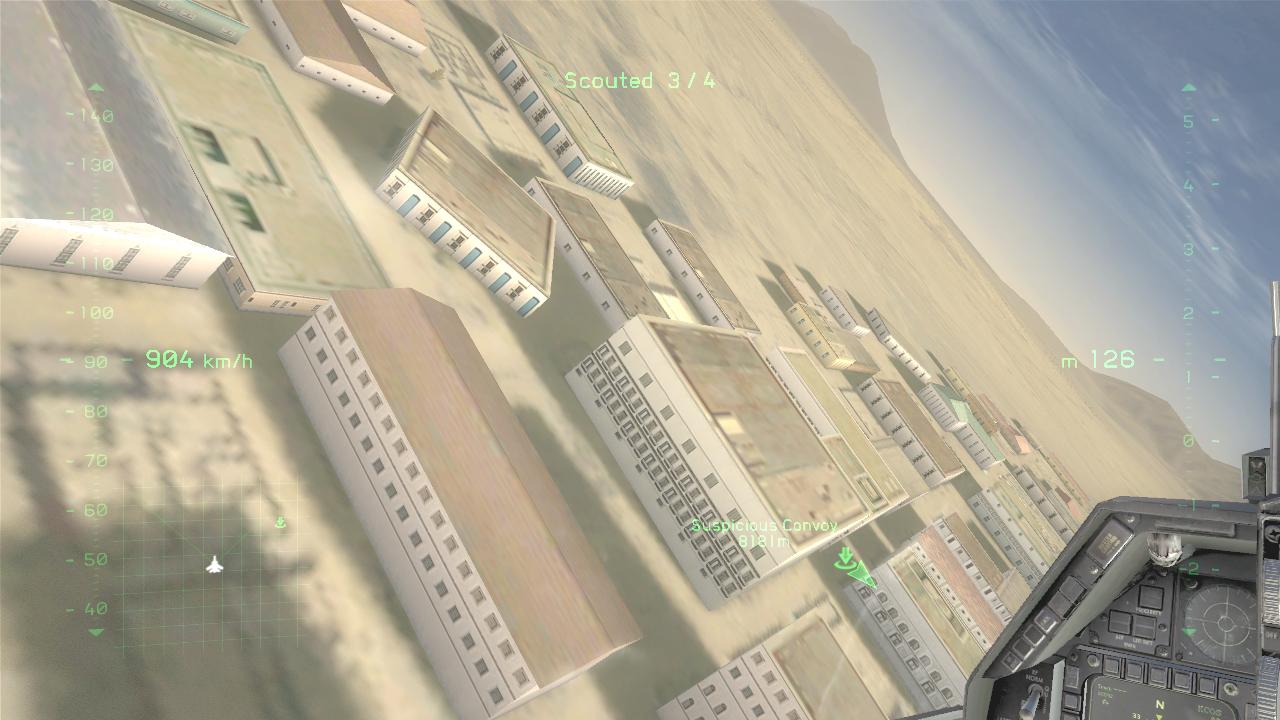A vibrant digital image appears to be a screenshot, potentially from a video game. The scene showcases a landscape filled with numerous simplistic buildings, predominantly rectangular with flat roofs, resembling industrial land structures. The buildings are tan in color with minimal design, each featuring a few windows. Interestingly, a few of these structures deviate from the norm, possessing sloped roofs akin to barns or silos.

Overlaying this background is a series of graphics, including notable numerical indicators such as "904 KM/H" and "M126." Additionally, there's text that reads "scouted 3/4," adding to the game's informational overlay. The composition of the shot is distinctly skewed, captured at a wild, almost sideways angle, enhancing the dynamic and somewhat disorienting perspective.

In the corner of the image, a discernible video game controller suggests that the image might be from an arcade game, likely a flight simulator given the presence of a substantial control interface. This deduction is reinforced by the grey console visible, typical of full-size arcade gaming setups.